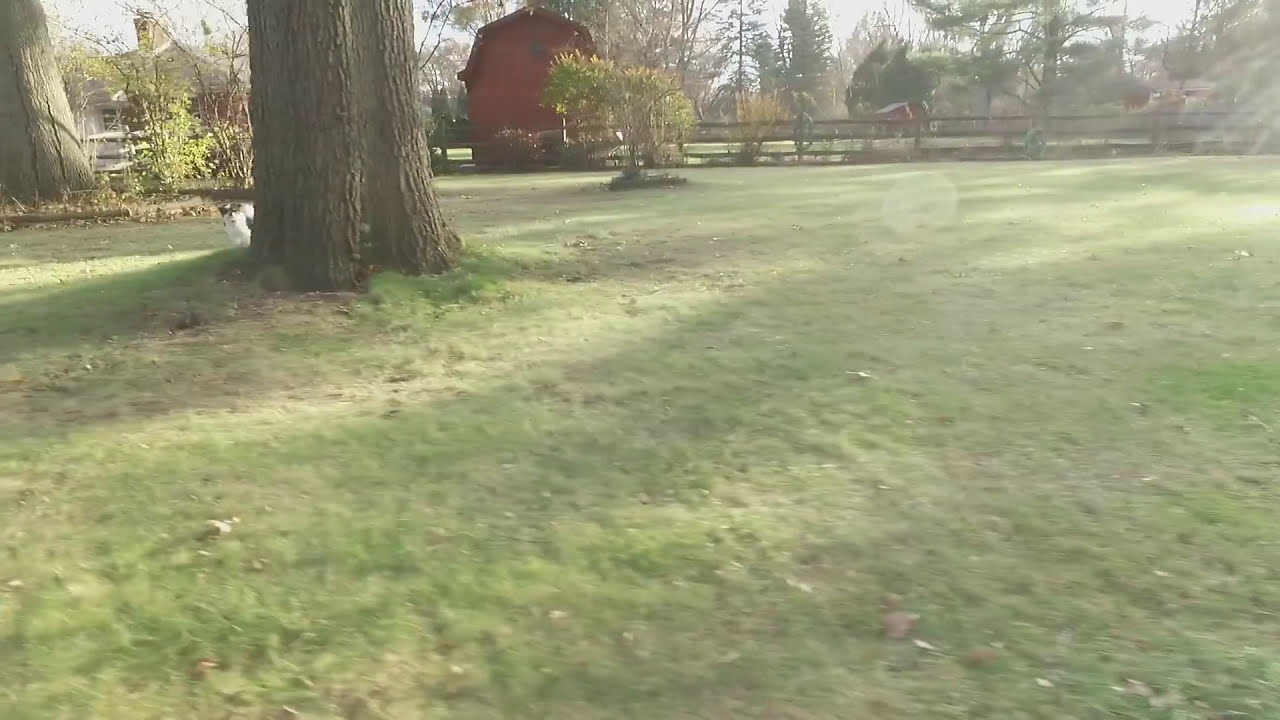The image is a color photograph taken on a bright sunny day, capturing a serene, park-like yard. The scene is slightly blurry but brimming with details. In the foreground, there is lush green grass interspersed with shadows. Dominating the left side are the trunks of two large trees, likely oak, with the lower portion visible. Peeking from behind the largest tree trunk is a small dog, mostly white with dark patches on its head, looking curiously toward the camera. Adjacent to the large tree, there's a smaller bush and a wooden fence stretching horizontally across the scene. Beyond the fence, a red barn stands prominently, and a partially obscured white house can be seen through some bushes in the top left corner. Trees in the background form a natural barrier, and the slivers of light gray sky peek through their leaves, adding depth to this representational realism photograph.